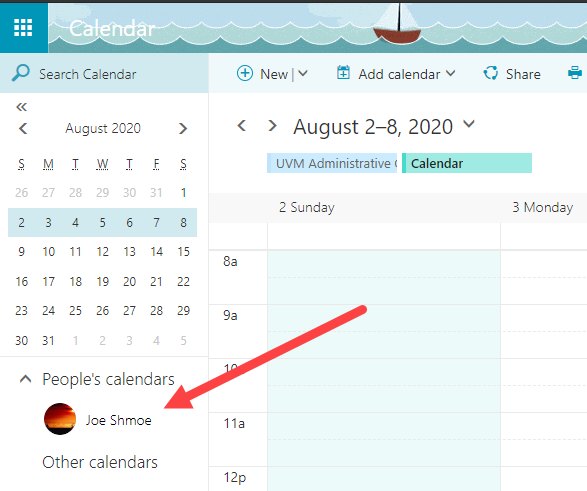The image features a stylized depiction of a beach scene positioned at the top. The beach is illustrated with two distinctly colored tiers of waves: the first wave being a light teal, followed by the second wave in a sea green hue. Both waves are accentuated with white outlines. Above the waves, the sky is depicted with a few scattered clouds in the center-right area. A sailboat with a white top and brown base leisurely floats on the water.

To the left of the scene, the word "calendar" is displayed in a basic sans serif white font. Adjacent to this text, nine white squares are arranged to form a larger square, set against a deep teal background. Beneath this visual, a search option is available, indicated by a teal magnifying glass icon, beside which the words "search calendar" are written in black.

The main section of the image displays a calendar set against a white background, indicating the month of August 2020. At the top of the calendar, there are navigation arrows: two arrows for changing the view, and beside the August 2020 title, left and right arrowheads for scrolling through the months. The days of the week are abbreviated as SMTWTFS, and the calendar spans from July 26th to September 5th. The grid is delineated by a thin gray border.

Below the calendar grid, on the left side, an upward-pointing arrowhead labeled "people's calendars" is visible, accompanied by an icon resembling a sunset, representing an account. Next to this icon is the name Joe Schmo. Further down, an "other calendars" section is identified, with a bold, red arrow pointing to Joe Schmo's calendar, extending from the 9 a.m. timeslot on August 2nd to August 8th.